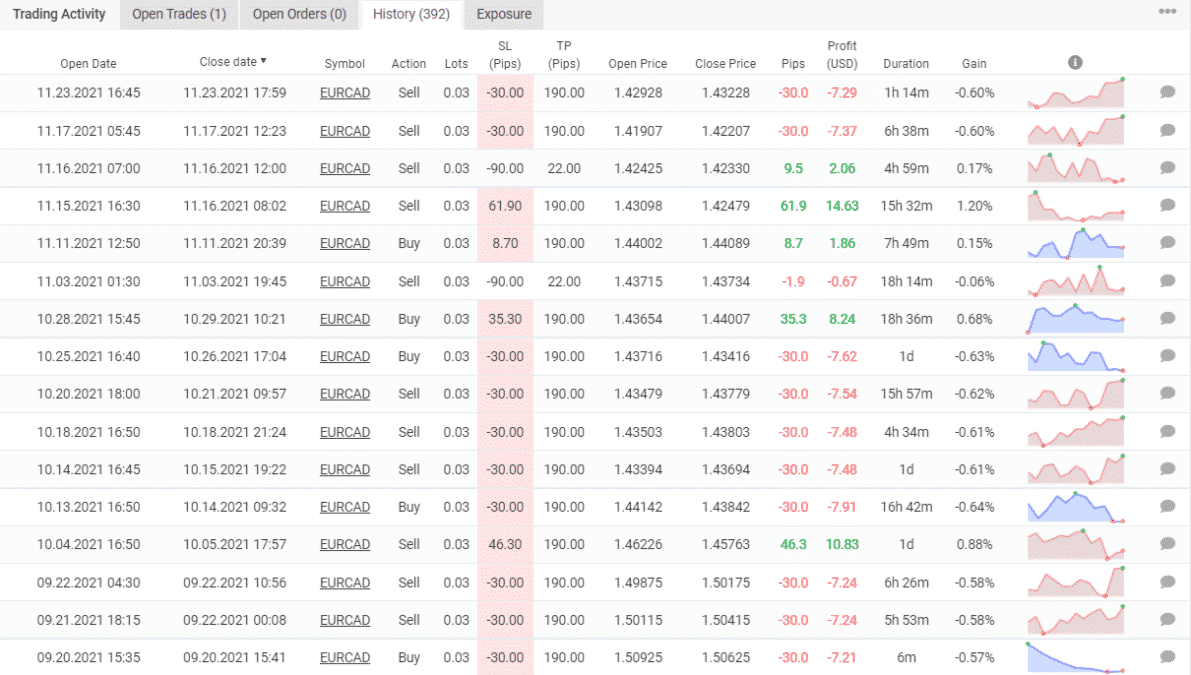**Detailed Descriptive Caption:**

The image appears to be a detailed screenshot of a trading platform's interface. The layout includes multiple tabs at the top: "Open Trades" (displaying '1' in parentheses), "Open Orders" (showing '0' in parentheses), "History" (marked with '392'), and "Exposure". These tab labels are grey, with the exception of the active "Trading Activity" tab, highlighted in white. 

To the right of these tabs is a grey band featuring a vertical ellipsis (three dots). Below this header, the interface displays a comprehensive table detailing various trading metrics. The table includes multiple columns: 

1. **Open Date**: Listing dates and times, starting with "11-23-2021, 1645".
2. **Closed Date**: Featuring corresponding close times.
3. **Symbol**: Mostly featuring "EURCAD" as the traded currency pair.
4. **Action**: Indicating "Buy" or "Sell" actions.
5. **Lots**: Quantity sizes, predominantly "0.0" but some entries are "0.5".
6. **Pro**: Contains highlighted numbers, such as "50", with some highlighted in peach.
7. **Pips**: Showing numerical values.
8. **Open Price**: A list of entry prices.
9. **Closed Price**: A list of exit prices.
10. **Pips (again)**: Repeated numerical values, green for positive and red for negative movements.
11. **Profit**: Numerical values, with positive amounts in blue and negative amounts in red.
12. **Duration**: Provided in hours and minutes.
13. **SAM**: Though it is too small to read clearly.
14. **Tiny Graphs**: Red or blue graphs representing trade movements.
15. **Circular Buttons**: Located to the right of each row.

Overall, the interface is optimally designed to present a summary of past trades, detailing each trade's performance metrics and outcomes.